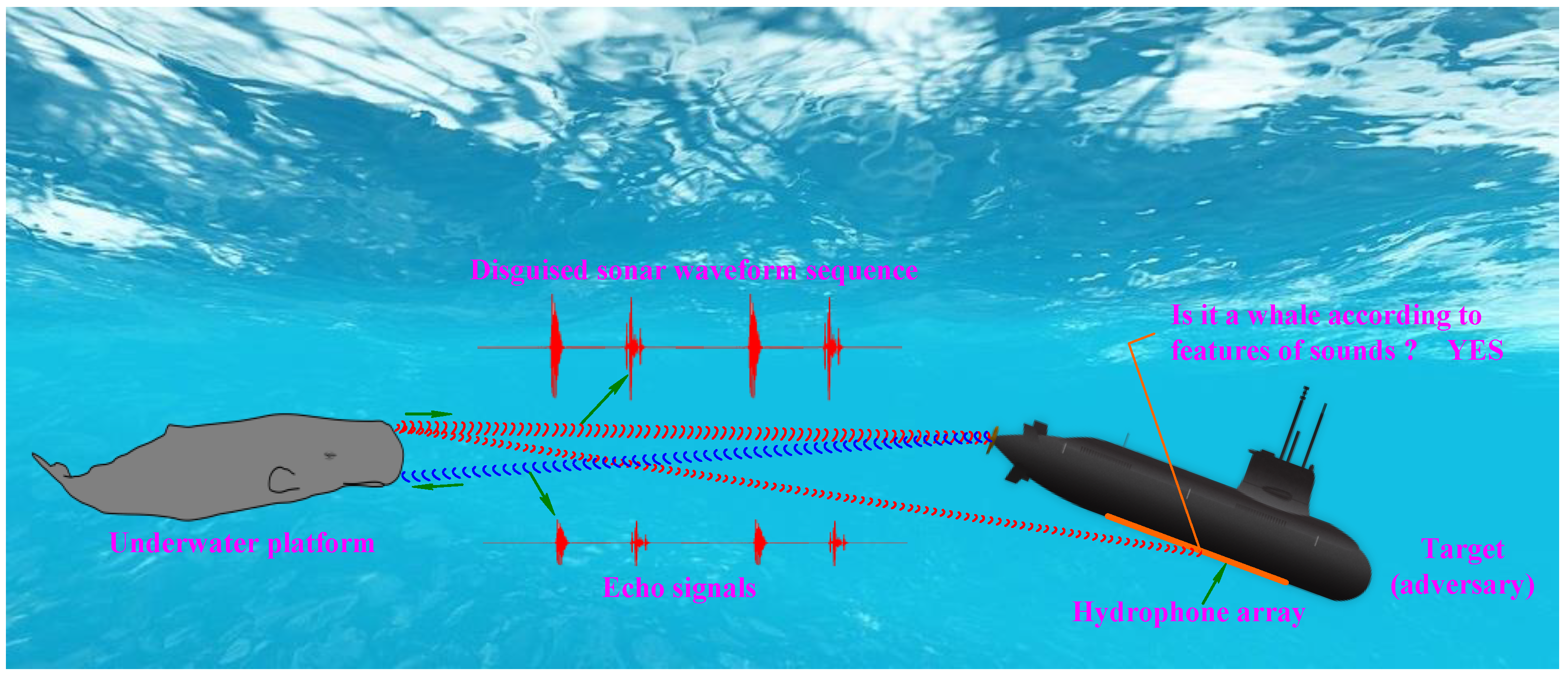The image is an undersea diagram in shades of blue, depicting light reflecting on water at the top. The scene showcases various underwater elements labeled in pink text. A hand-drawn gray whale is situated on the left side of the diagram, with the word "underwater" written beneath it. To the right, there is a gray submarine in the process of diving, labeled "hydrophone array" and "target adversary" to its right. Between the whale and the submarine, red arrows and sonar sound wave lines are shown, symbolizing signals. The diagram also includes text such as "disguised sonar wavelength sequences" and "echo signals" in pink, with red and blue arrows pointing from the whale to the submarine. A key query, "Is it a whale according to features of sounds?" is posed above the submarine, with the answer "yes" provided. The background is a clear, crystal blue, suggestive of ocean water, with additional water ripples and waves visible at the top.